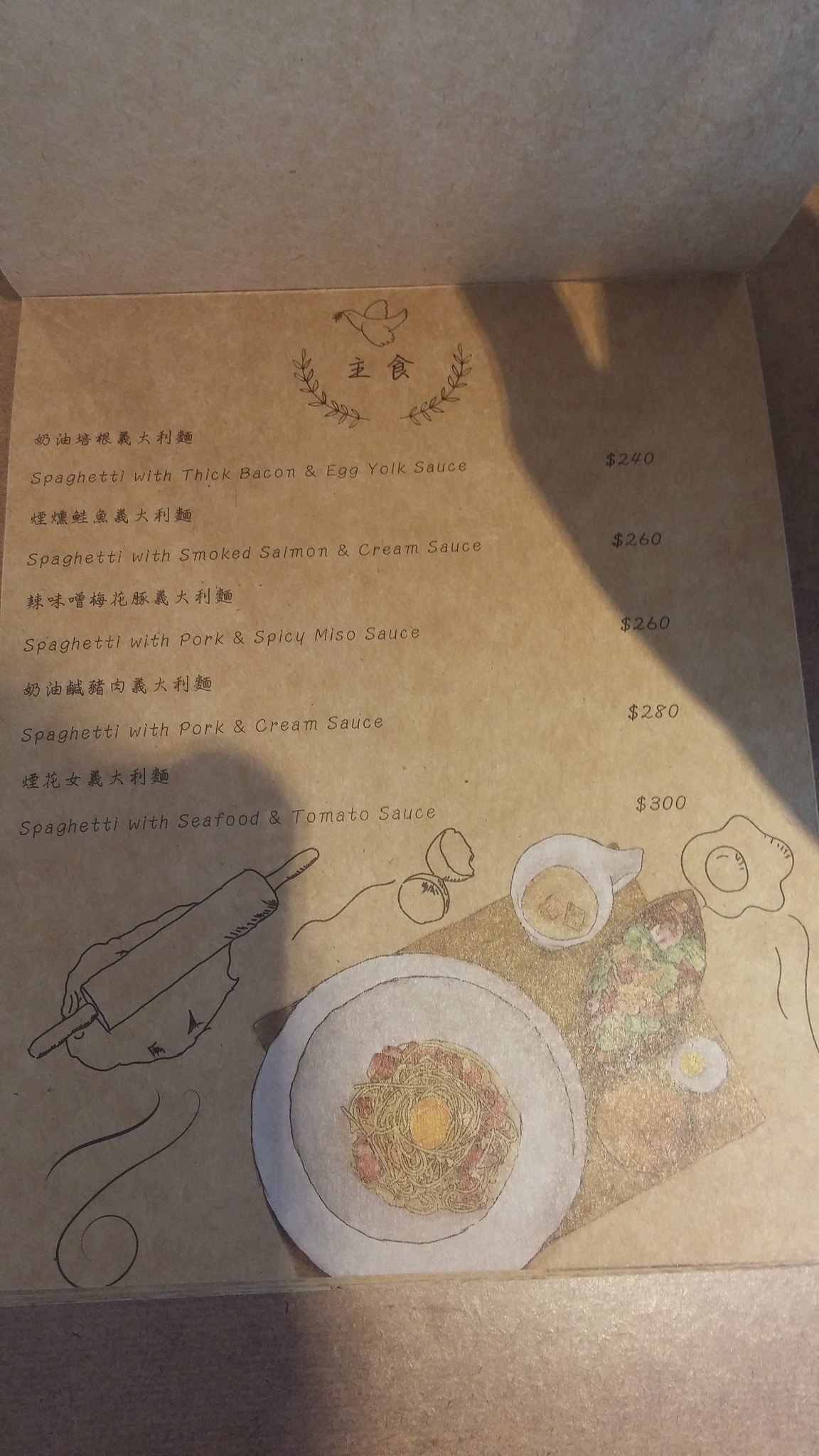The image captures a color photograph of what appears to be a restaurant menu, not a grave plaque as initially assumed. The menu is printed on parchment-colored paper, giving it an antique feel. At the top of the menu, there is an artistic depiction of a peace dove holding an olive branch in its beak. Beneath the dove are Chinese characters and illustrations of small laurel or olive branches, adding to the decorative elements.

The menu itself is divided into sections with both Chinese and English text, although the specifics of the items are not fully legible. Illustrations line the bottom of the menu, including a rolling pin rolling out dough, what appears to be a cracked egg, and a fried egg situated to the right. In the center, there is a colorful illustration of a bowl, possibly containing soup, and to its right, a depiction of a fish on a serving platter, adding a vibrant touch to the otherwise simple line art.

The menu is placed on a shiny tabletop, which is evident from the glistening surface seen at the bottom of the image. Shadows cast across the bottom left and top right corners, contrasted by a bright light illuminating the lower part of the menu. 

The menu lists five items, described in both Chinese and English, though the text is difficult to read. Among the discernible items are dishes that mention spaghetti, smoked salmon, and pork in a cream sauce, accompanied by seemingly high prices to the right of each description.